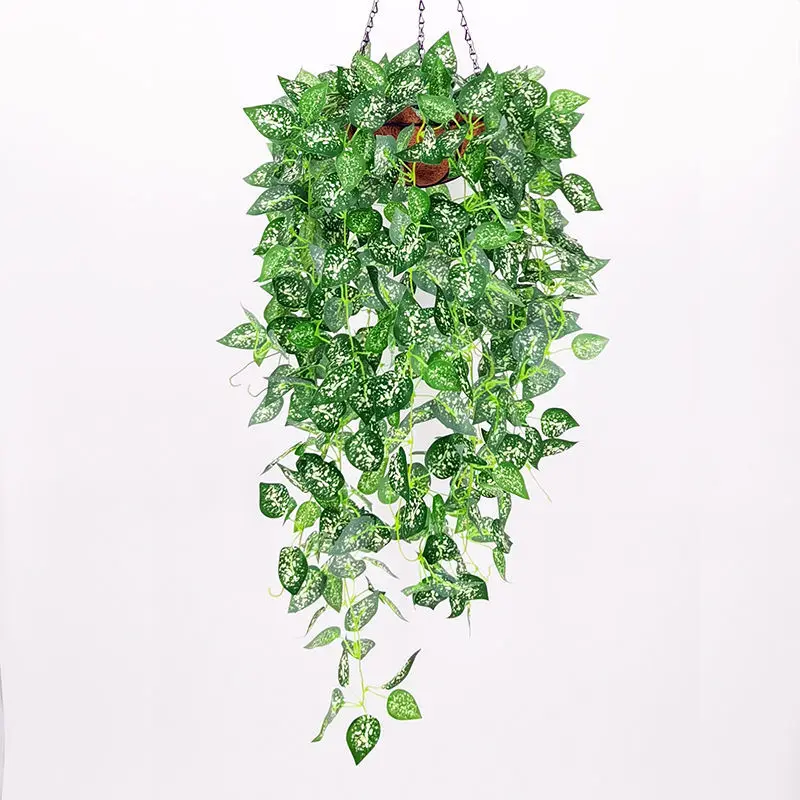This image depicts a vibrant ivy plant cascading from a terracotta-colored hanging planter, supported by three silver chains. The planter, adorned with a broader rim, is suspended from above, captured only about a foot down from its hanging point. The ivy, characterized by its teardrop-shaped variegated leaves, features a striking green hue with white speckles. The lush foliage spills over the planter’s edge, gradually tapering to a single leaf at the bottom, creating a graceful, draping effect. The plant’s vine-like tendrils and varied leaf density contribute to its flowing appearance, evocative of a creeping Charlie, as the branches and leaves are elegantly pulled down by gravity. There is no text visible in this photo.